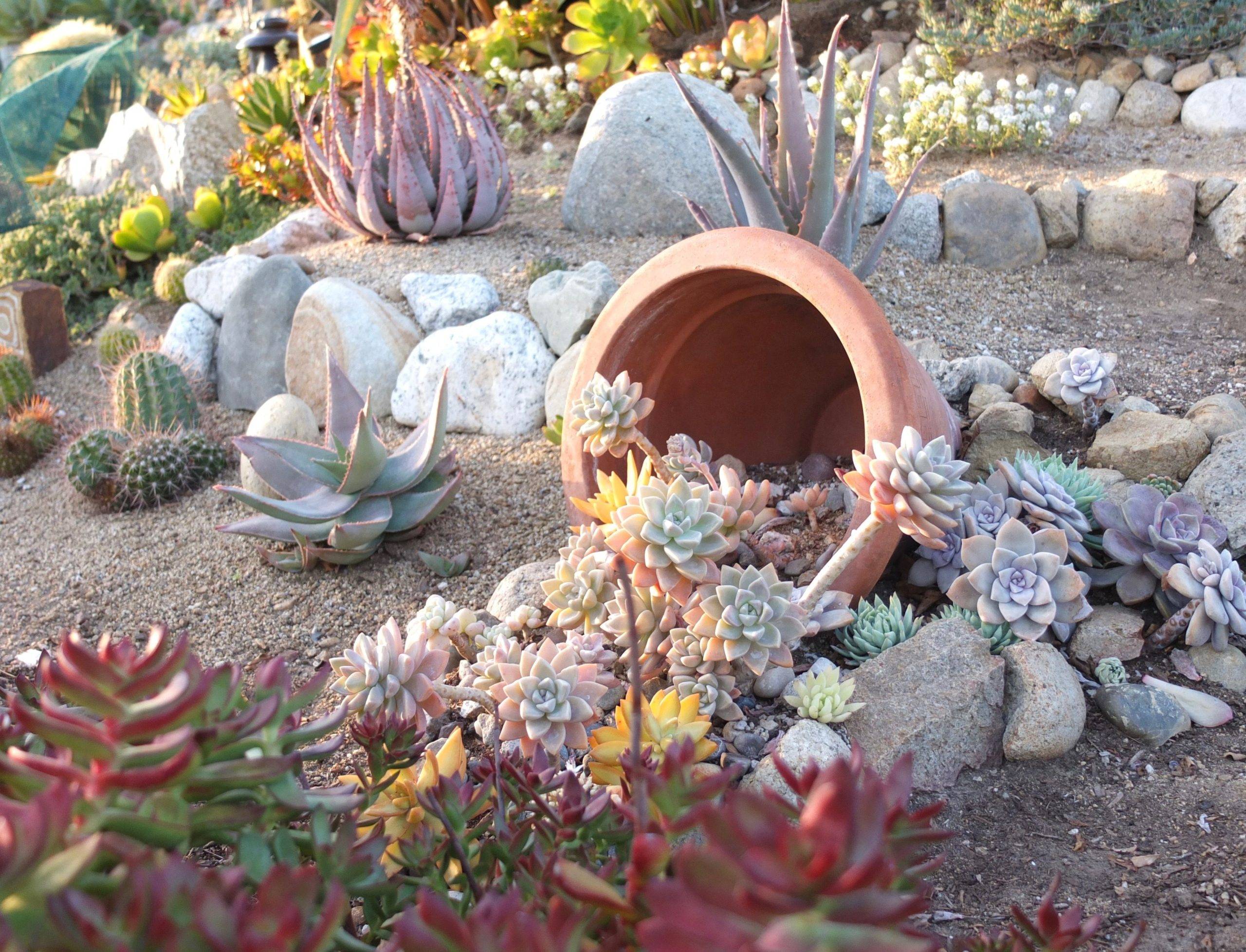This is a detailed color photograph depicting an intricately designed garden scene filled with various types of succulents and cacti. The landscape is structured with sandy soil and layers of large rocks forming tiered steps. At the center of this outdoor oasis lies a terracotta pot tipped over decoratively, from which small succulent plants are sprawling outwards. The garden showcases a variety of flora that are adept at retaining water, presenting a mixture of textures and colors.

In the foreground, some green and red cacti are slightly out of focus, foregrounding a vibrant scene. To the left of the pot, there are green cacti with pointy projections, and nearby a spiky green cactus adds to the diversity. The garden is segmented into three layers of height, with the lowest tier displaying dark soil and more diminutive plants. The middle tier offers plants with long, purplish bladed leaves, and the uppermost tier consists of smaller plants clustered together, adding richness to the rocky background. A distinctive line of stones meanders from the lower right, curving upwards and forming a boundary around this lush display, encapsulating pink-hued cacti with whitish-pink petal-like projections. The overall scene is a harmonious blend of natural elements, showcasing a variety of plants thriving in a beautifully arranged, tiered garden space.